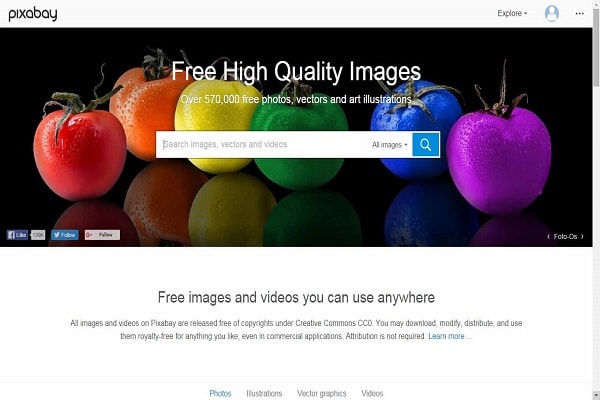This is a horizontally-oriented web page from the website Pixabay. The page features a vibrant, eye-catching banner approximately two inches in height. Central to the image is a white search box, displaying the prompt "Search images, vectors, and videos" in gray text. A dropdown menu adjacent to the search box is currently set to search "all images."

The background of the banner showcases a vivid photograph of six pieces of fruit, each in different colors: a red strawberry, an orange, a yellow fruit, a green fruit, a blue fruit, and a purple fruit. All fruits are similarly sized and have stems at the top. They rest on a glossy black surface that reflects their colorful images, with the rest of the background remaining solid black to highlight the fruits.

Above the search box, in bold white text, the page proclaims "Free high-quality images." Below this, in smaller white text, it mentions "Over 570,000 free photos, vectors, and art illustrations." The colorful and vibrant arrangement of the fruits, combined with the clear and straightforward search functionality, encapsulates the essence of Pixabay as a resource for high-quality, free visual content.